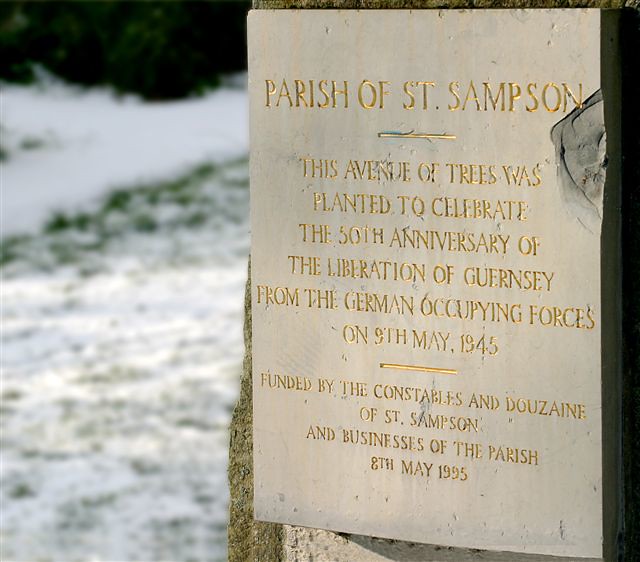The image features a concrete plaque affixed to the corner of a historic building. The plaque is dedicated to commemorating the 50th anniversary of the liberation of Guernsey from German occupying forces on May 9th, 1945. The plaque, with its white background and gold engraving, reads: "Parish of St. Samson. This avenue of trees was planted to celebrate the 50th anniversary of the liberation of Guernsey from the German occupying forces on May 9th, 1945, funded by the constables and the Douzaine of St. Samson and businesses of the parish, May 8th, 1995." The surrounding environment is blurry, but it appears to be snowy, adding a serene backdrop to the commemorative plaque. The text on the plaque is engraved in a manner reminiscent of headstones found in cemeteries, and the capitalized letters convey its formal significance.